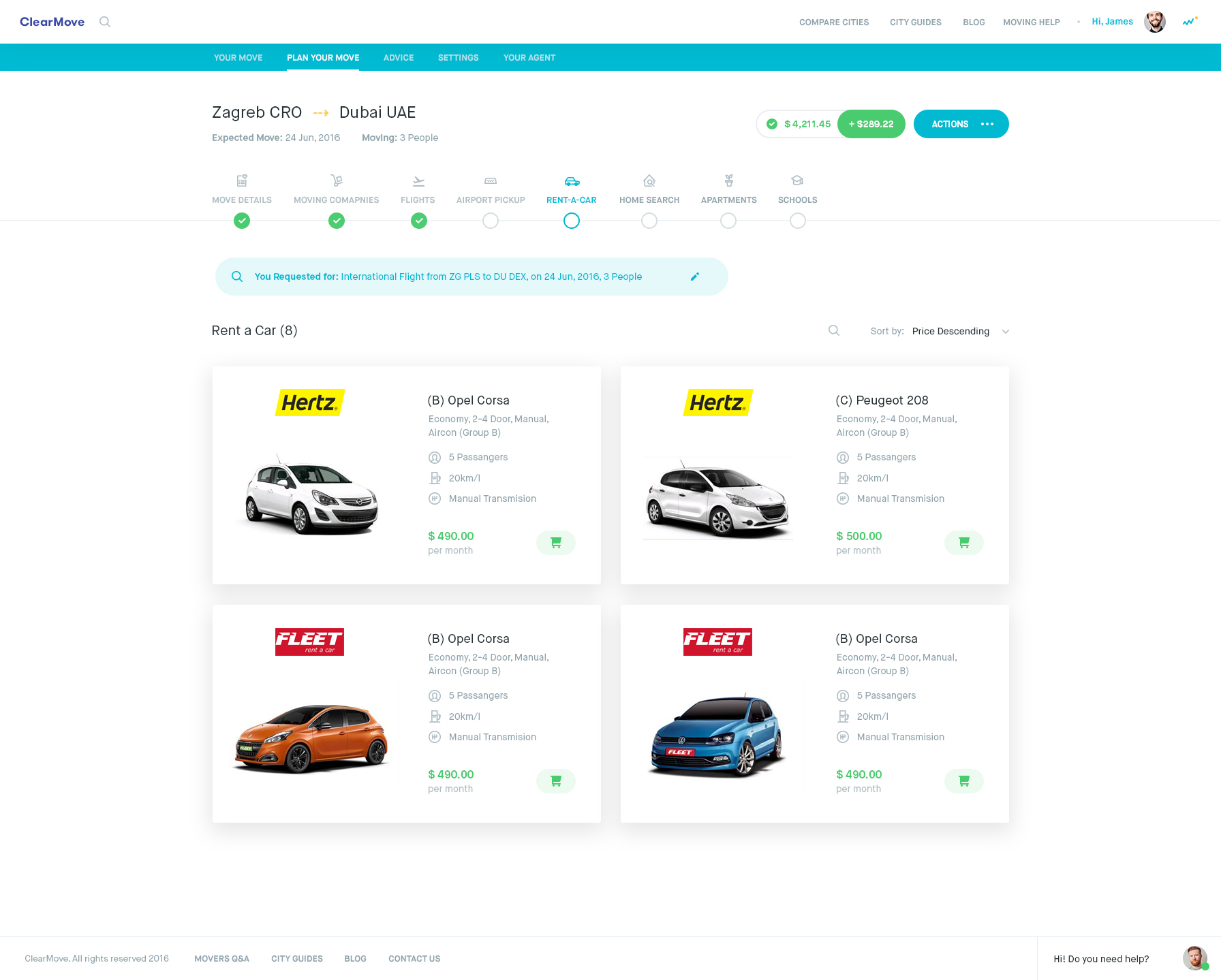This is a detailed screenshot of a Hertz car rental website. The page is densely populated with various sections and textual elements. Despite zooming in, the text remains indecipherable.

1. **Top Left Corner:** Displays the Hertz logo prominently.
2. **Top Right Corner:** Contains multiple headings, supplemented by a small icon.
3. **Blue Banner:** Features a blue rectangular banner with white text headings.
4. **Central Section:** Indicates travel details from "Zagreb, CRO" to "Dubai, UAE,” suggesting a rental scenario linked to travel.
5. **Numerous Headings:** Below the travel details, there are a series of headings. Some of these are accompanied by check marks within green circles, while others are marked by empty circles.
6. **Action Buttons:** Shows a green button and a blue button, presumably for interactive actions.
7. **Search Bar:** A blue search bar contains some unreadable text.
8. **Car Display Section:** 
    - Shows multiple Hertz logos, each illustrating a different car model with accompanying details.
    - First depiction: Hertz logo in a yellow rectangle with black text, adjacent to a white car and associated information.
    - Second depiction: Similar Hertz logo with another white car and its information.
9. **Fleet Section:**
    - First entry: The word "Fleet" within a red box and an orange car displayed next to its details.
    - Second entry: The word "Fleet" again in a red box, adjacent to a blue car with its associated information.

Overall, the screenshot exemplifies a well-organized webpage meant to facilitate straightforward car rental transactions, despite the illegible text.